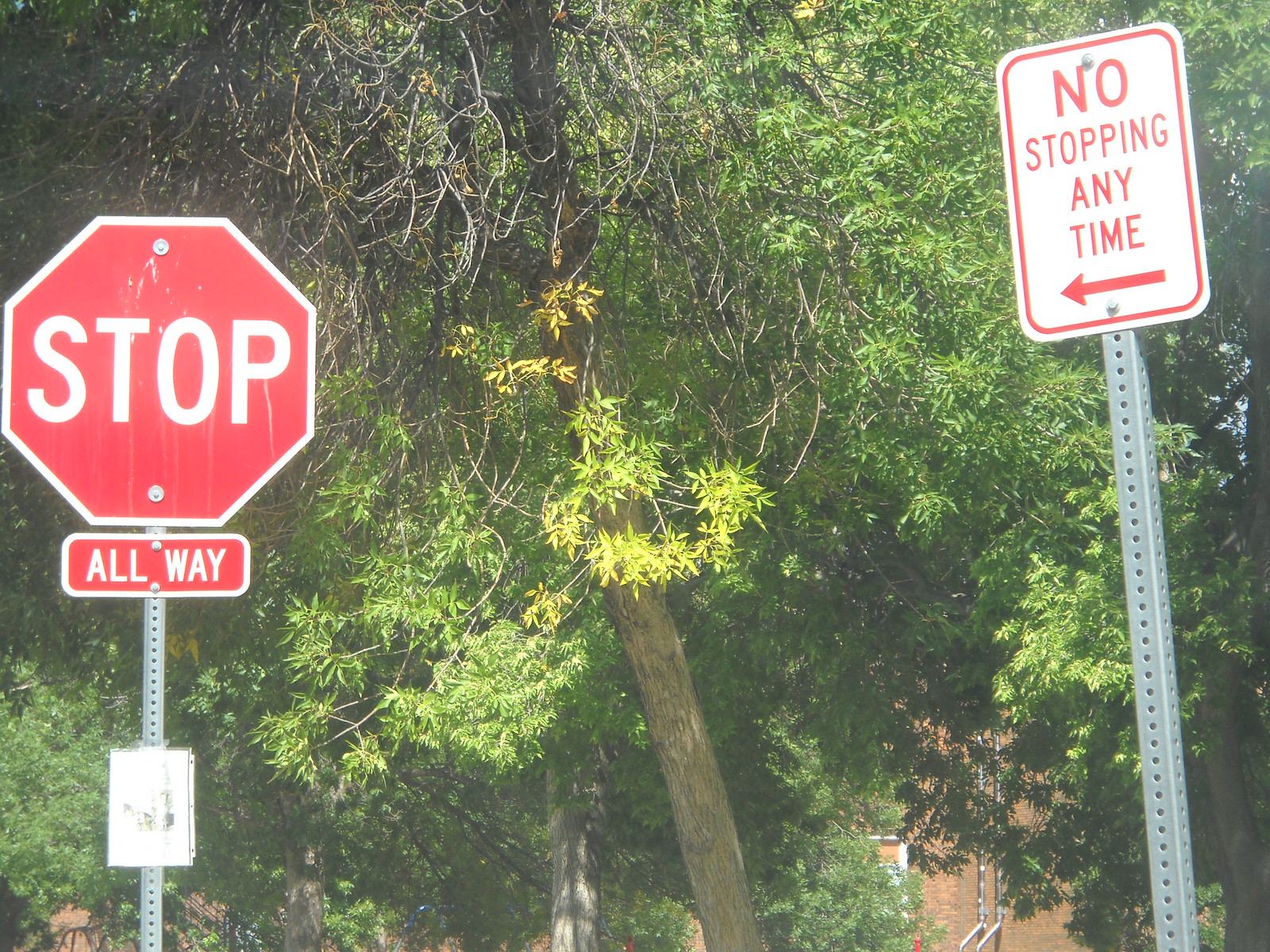The photograph, taken outside on a bright, slightly overexposed day, depicts a street scene dominated by two prominent street signs and a tree set against a brown stone building. The tree, with its vividly lit green leaves, runs diagonally through the center of the image. On the left side, a traditional red octagonal stop sign with bold white letters is affixed to a perforated metal pole; underneath it is a red rectangular "all way" sign, indicating a multi-directional stop at the intersection. Additionally, there appears to be a community-taped laminated white paper on the pole, though the text is indistinguishable. On the right side of the image, another perforated metal pole supports a white rectangular "no stopping any time" sign bordered and lettered in red, with a leftward-pointing arrow directing towards the central tree and stop sign. The street scene, framed by the contrasting colors of the signs and greenery, suggests a typical neighborhood setting in the United States.